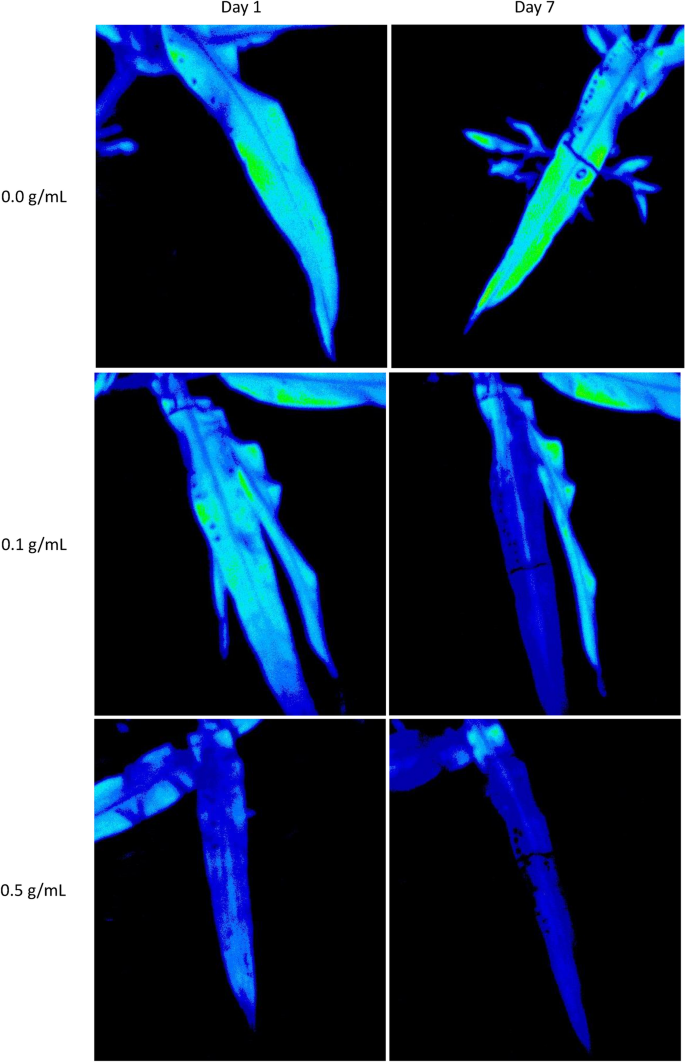The image presents a six-panel collage showcasing the progression of plant leaves over a period of seven days, highlighted in fluorescent ultraviolet colors of neon blue and green against a black background. The panels are arranged in three rows and two columns, with each row corresponding to different concentrations: 0.0 g/mL, 0.1 g/mL, and 0.5 g/mL. The top row is labeled "Day 1" on the left and "Day 7" on the right, indicating the time progression for each concentration. Each panel features elongated leaves, typically comprising two to three per section, with a distinct dividing line in the center. The leaves exhibit a striking transformation: starting with a vibrant mix of neon blue and green, gradually turning more predominantly blue by the second panel, and showing signs of deterioration and deep blue hues by the final set. This visually detailed sequence captures the morphological changes and possibly the effects of different treatments over time.